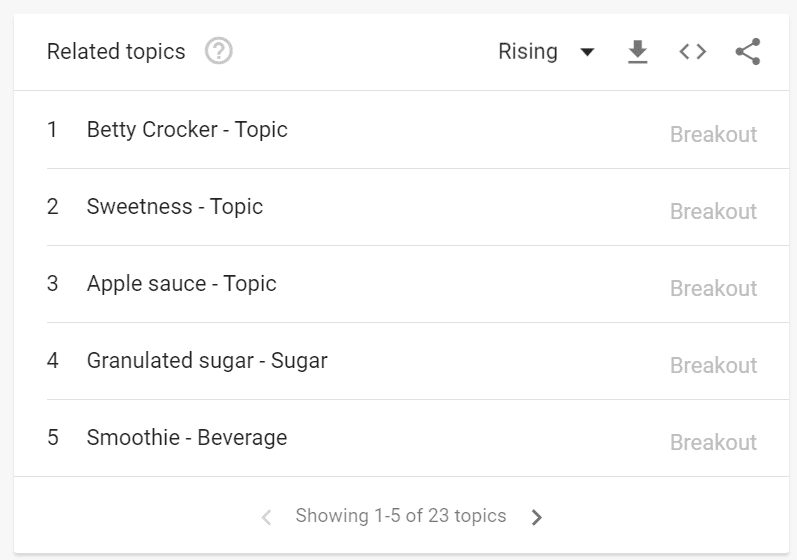The image depicts a structured user interface framed by a gray border. At the very top, a title reads "Related Topics," accompanied by a question mark enclosed within a gray circle to the left. Adjacent to this, on the right, is the word "Rising" next to a dropdown menu indicated by a downward-pointing arrow. Further along the same row are several functional icons: a download symbol represented by a downward arrow above an underline, a left-facing less than symbol, a right-facing greater than symbol, and an interconnected chart icon depicting two circles connected by a diagonal line, with one circle pointing up and the other pointing down.

Beneath this, a thin gray line separates the top row from the list of topic breakouts. The first entry starts with:

1. "Betty Crocker - Topic Breakout"

Following this, separated by another thin gray line, are additional entries:

2. "Sweetness - Topic Breakout"
3. "Applesauce - Topic Breakout"
4. "Granulated Sugar - Sugar Breakout"
5. "Smoothie - Beverage Breakout"

Below the fifth entry is a control panel with the less than symbol "<" showing "1-5 of 23 topics" followed by the greater than symbol ">".

Each section is clearly delineated by thin gray lines, ensuring a neat and organized appearance.